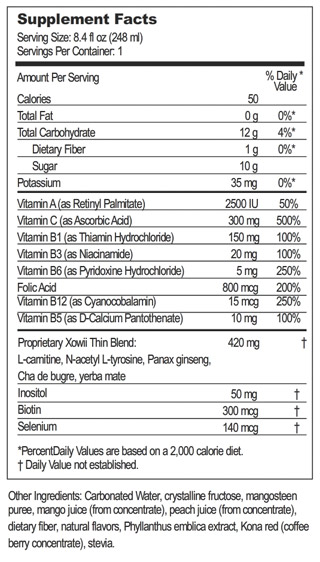The image displays a "Supplement Facts" label set against a white background with a black border. The label is organized within a tall, rectangular box, lined with horizontal black lines. At the top, it reads "Supplement Facts," followed by details about the serving size (4.4 ounces or 4.82 milliliters) and the amount per serving. Nutritional information per serving includes 50 calories, 0 grams of total fat, 12 grams of carbohydrates (4% DV), 1 gram of dietary fiber, 10 grams of sugar, and 35 milligrams of potassium. The label extensively lists vitamins and minerals, including Vitamin A (250 IU, 50%), Vitamin C (300 milligrams, 500%), Vitamin B1 (150 milligrams, 100%), Vitamin B3 (20 milligrams, 100%), Vitamin B6 (5 milligrams), Folic Acid (800 milligrams, 200%), Vitamin B12 (15 milligrams, 250%), and Vitamin B5 (10 milligrams, 100%). A proprietary blend of 420 milligrams features ingredients such as L-Carnitine, L-Tyrosine, and Panax Ginseng, along with additional elements like Biotin, Inositol, and Selenium (440 milligrams). The label notes that the percent daily values are based on a 2,000-calorie diet, and some nutrients do not have established daily values. Below the main box, the label lists other ingredients, including carbonated water, crystalline fructose, mango and peach juices from concentrate, dietary fiber, natural flavors, and stevia.